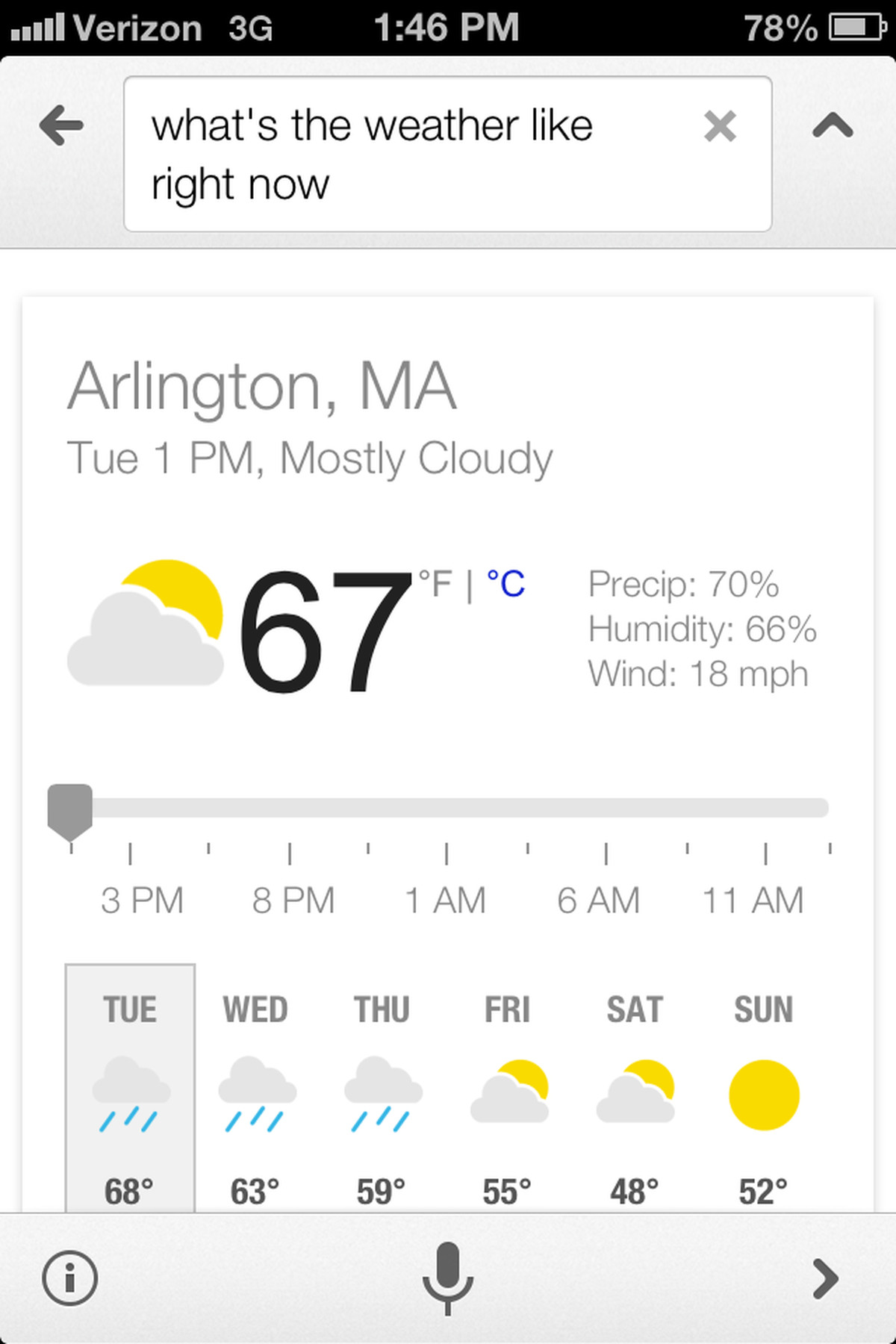**Detailed Descriptive Caption:**

This screenshot captures the interface of a smartphone displaying weather information. At the top of the image, the status bar shows the phone signal as Verizon 3G, the time as 1:46 PM, and the battery level at 78%. Below the status bar, there is a white query box against a gray background with the text "What's the weather like right now?" Inside this box, there is an 'X' icon for closing it, as well as arrows pointing left and up.

The main section of the screenshot provides detailed weather information for Arlington, MA. It indicates that it is Tuesday at 1 PM with mostly cloudy conditions and a temperature of 67 degrees Fahrenheit. Additional weather details include a 70% chance of precipitation, 66% humidity, and winds blowing at 18 miles per hour.

Further down, there's a sliding graph summarizing the weather forecast for the coming days. Specifically, for Tuesday, it notes rain at 3 PM with a temperature of 68°F, and at 8 PM the temperature drops to 63°F with continued rain into Wednesday. The forecast for the rest of the week is as follows:
- Wednesday: Rain and 63°F.
- Thursday: Rain and 59°F.
- Friday: Partly sunny with a high of 55°F.
- Saturday: Partly sunny and 48°F.
- Sunday: Sunny with a high of 52°F.

The bottom bar of the screen includes various functional icons such as a microphone and an arrow pointing to the right.